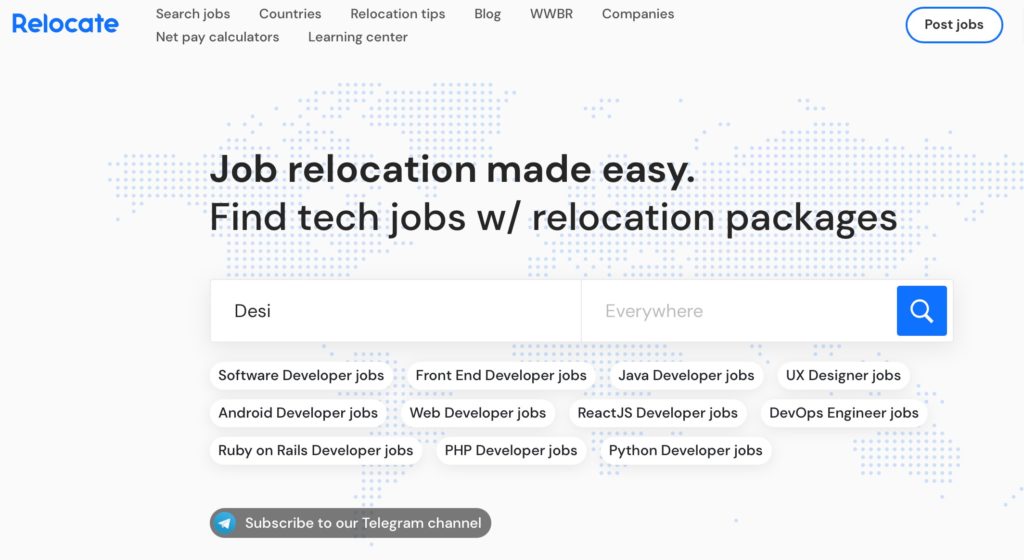The image features a clean and simple webpage design with a predominantly white background accented by subtle light blue dots arranged to resemble the continents of the Earth. Overlaying this backdrop, the headline in bold black letters reads, "Job Relocation Made Easy." Beneath the headline, a subheader states, "Find tech jobs with relocation packages."

Located underneath the subheader is a search bar that prominently displays the placeholder text "DESI" and "everywhere" alongside a search magnifying glass icon. Following the search bar, several oval-shaped buttons are arranged in multiple rows, each listing various tech job categories:

- The first row includes buttons labeled "Software Developer Jobs," "Front End Developer Jobs," "Java Developer Jobs," and "UX Designer Jobs."
- The second row features "Android Developer Jobs," "Web Developer Jobs," "React.js Developer Jobs," and "DevOps Engineer Jobs."
- The third and final row lists "Ruby on Rails Developer Jobs," "PHP Developer Jobs," and "Python Developer Jobs."

At the bottom of the page lies a prominent elongated gray oval button with a red circle and an arrow icon inside it. This button is accompanied by the text, "Subscribe to our Telegram channel," inviting users to stay updated on the latest job offerings.